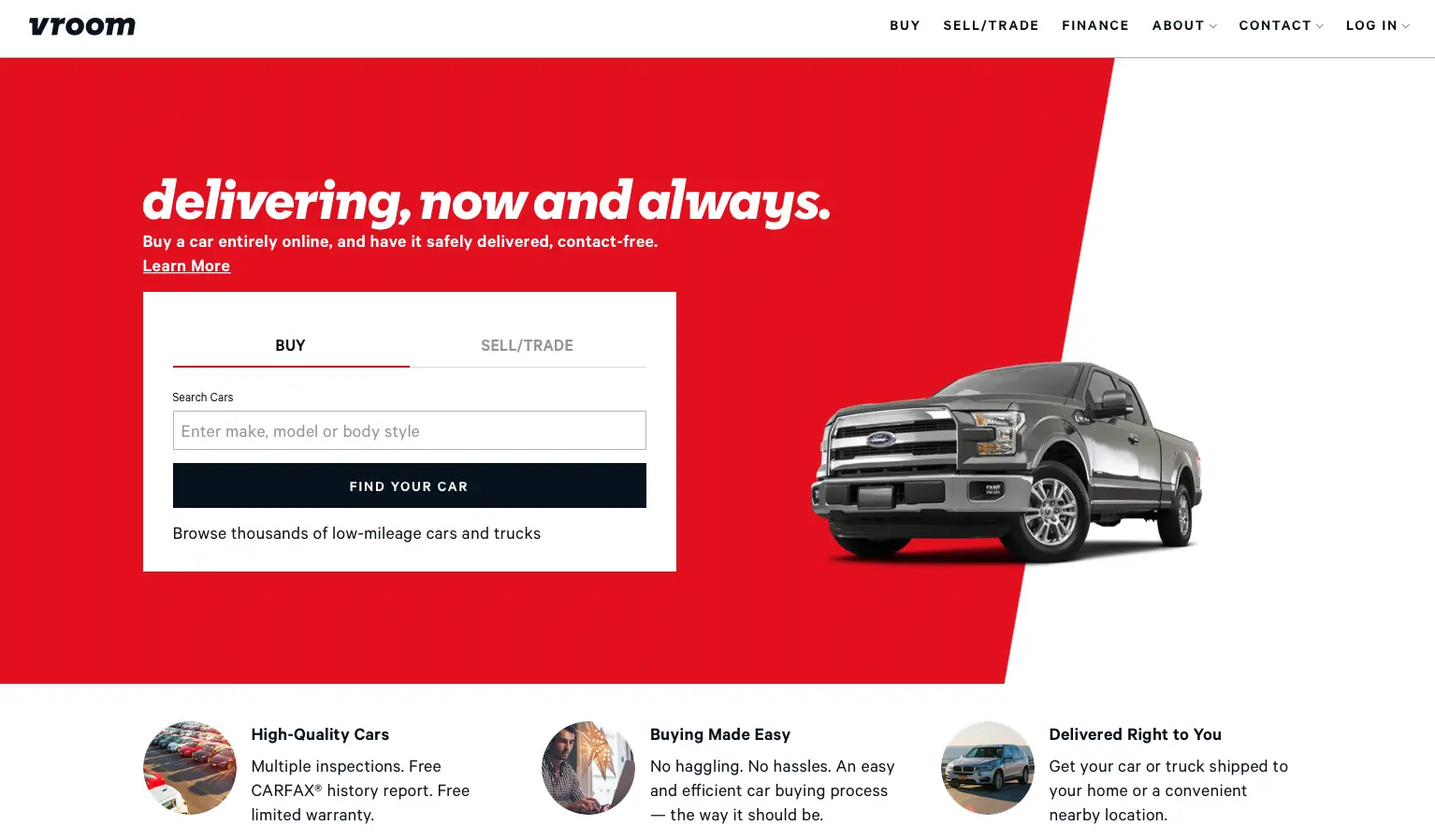The image showcases a car dealership website, characterized by a sophisticated yet straightforward layout. Dominating the top left corner is the brand name "VROOM," presented in bold black text. At the top right corner, essential navigation links are displayed, including "LOGIN," "CONTACT," "ABOUT," "FINANCE," "SELL & TRADE," and "BUY."

Central to the image, slightly off-center to the right, is a striking visual of a black truck. The vehicle is slightly tilted to the left, capturing the gleam of reflective light on its left side. The truck's front is adorned with three prominent metal grilles, adding to its robust appearance.

On the left side of the truck, bold and captivating words read "DELIVERING NOW AND ALWAYS." Beneath this statement, a white, rectangular interactive section offers navigation options. Here, the word "BUY" is highlighted with a red horizontal line beneath it, while "SELL & TRADE" appears to the right.

At the bottom of this section, a prominent rectangular search box awaits user input, featuring the prompt "ENTER MAKE, MODEL, or BODY STYLE," guiding users to begin their vehicle search.